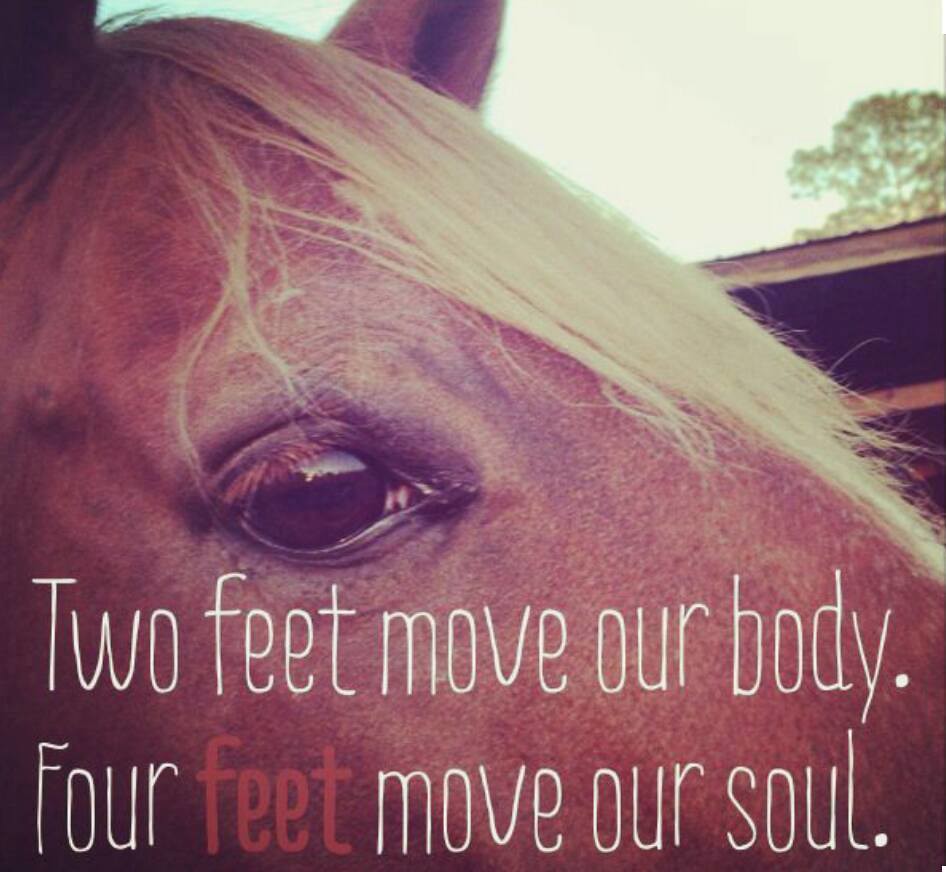This image depicts a close-up of a brown horse's head, with a particular focus on its large, reflective brown eye at the center. The horse's distinctive feature is its mane, which is strikingly much lighter than its coat, appearing almost blonde or white. The photo captures just the lower part of the horse's ears and does not include its mouth or nostrils. In the background, the sky appears desaturated and light green, with a tall tree and a partial view of a barn or shed, suggesting the horse's shelter. The image is overlaid with text in white, with a notable emphasis in red saying, "Two feet move our body. Four feet move our soul." This highlights the photographer's and possibly the viewer's emotional connection to horses, emphasizing their deep appreciation and love for these majestic creatures.